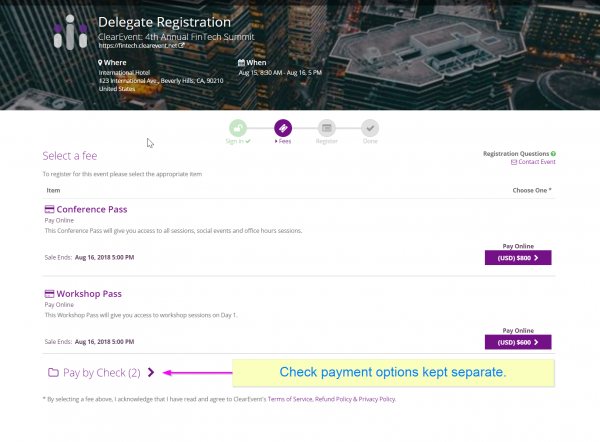The image displays a vibrant banner at the top featuring a modern cityscape with numerous tall buildings of varying sizes and heights. Dominating the foreground in bold white print, it reads "Delegate Registration," with the 'D' and 'R' capitalized. Beneath this, the text "ClearEvent" appears, formatted as one word with both the 'C' and 'E' capitalized.

Further down, a colon introduces the event title: "4th Annual FinTech Summit," with 'FinTech' presented as a single word, featuring a capital 'F' and 'T'. The website for additional information is provided below this title. The image then details the event's location and schedule, listing the address, dates, and times clearly.

The lower section of the image transitions to a white background, decorated at the top with small circles in varying colors: the first one green, followed by purple, and two gray circles. In purple print, the phrase "Select a Fee" is displayed, accompanied by a mouse pointer hovering nearby.

Underneath this section, the image outlines different registration options:
- "Conference Pass" to be paid online, with the sale end date prominently noted.
- A purple square featuring "Workshop Pass," also to be paid online, with the notation that the sale ends on August 16th at 5 p.m.
- An option "Pay by Check," indicated by a right-pointing arrow.

Accompanying this, a long left-pointing arrow explains that "Check Payment Options Kept Separate."